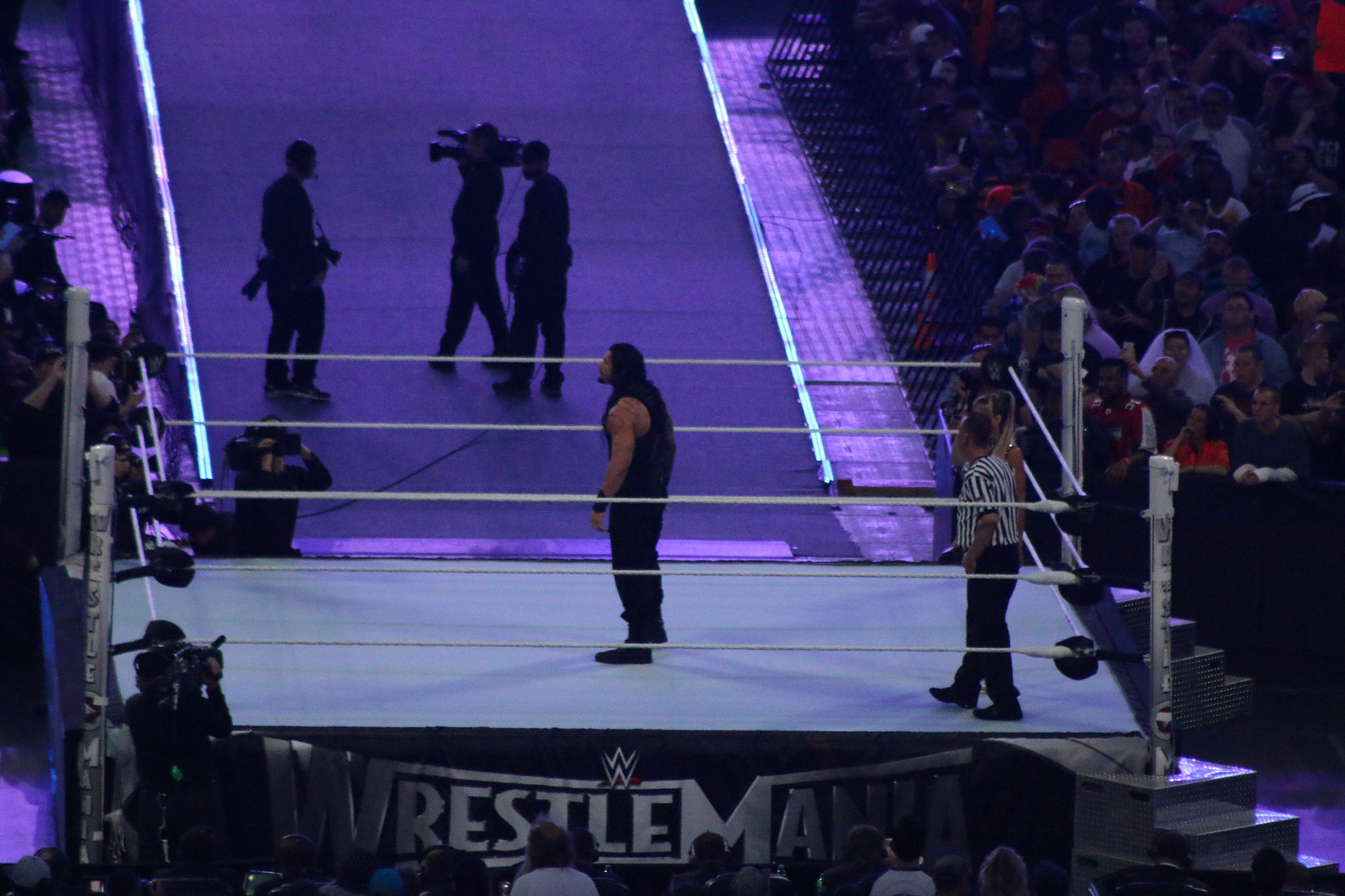This image captures an exhilarating moment from WrestleMania, a WWE professional wrestling event, taken from the perspective of someone in the stands. In the middle of the wrestling ring, a formidable wrestler with long black hair, dressed in a black tank top, pants, and shoes, stands menacingly, looking out into the crowd. The wrestling ring, adorned with the WrestleMania logo and surrounded by white boundary ropes, has a primarily light blue to slightly gray mat.

In the nearest right corner inside the ring stands a referee in a classic black and white striped shirt with black pants. Tucked next to the referee is a partially obscured blonde woman. The arena's ambiance is set by a dark, purplish lighting, bathing the scene with an anticipatory hue as if a match announcement is imminent.

Beyond the ring, a hive of activity unfolds with camera crews and photographers capturing every moment, positioned along the ramp—the entrance walkway highlighted by purple lights. Spectators fill both sides of the ramp, their heads visible as they eagerly take in the spectacle. The scene offers a glimpse into both the raw energy of the event and the orchestrated chaos behind the scenes.